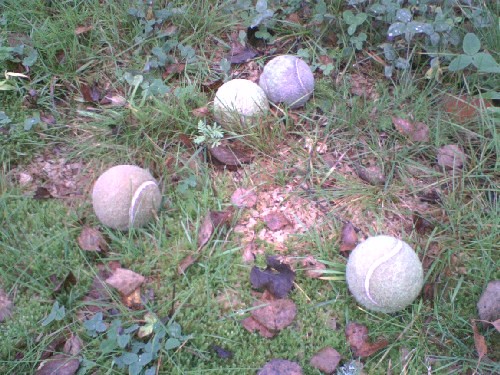This close-up image captures a neglected backyard scene featuring four heavily discolored and worn tennis balls scattered across a patchy expanse of grass. The grass varies in height and includes clover with white spots, as well as green and brown leaves, some almost blackened. Among the details, two pale gray tennis balls are positioned side-by-side in the upper center of the image, while the remaining two—one tan and one dark gray with a white spot—are spread apart, with one located in the lower left and the other in the lower right corner. In the upper right-hand corner, a small cluster of shrubs with three leaves adds to the natural disarray, hinting at the passage of time and lack of upkeep in this outdoor space.